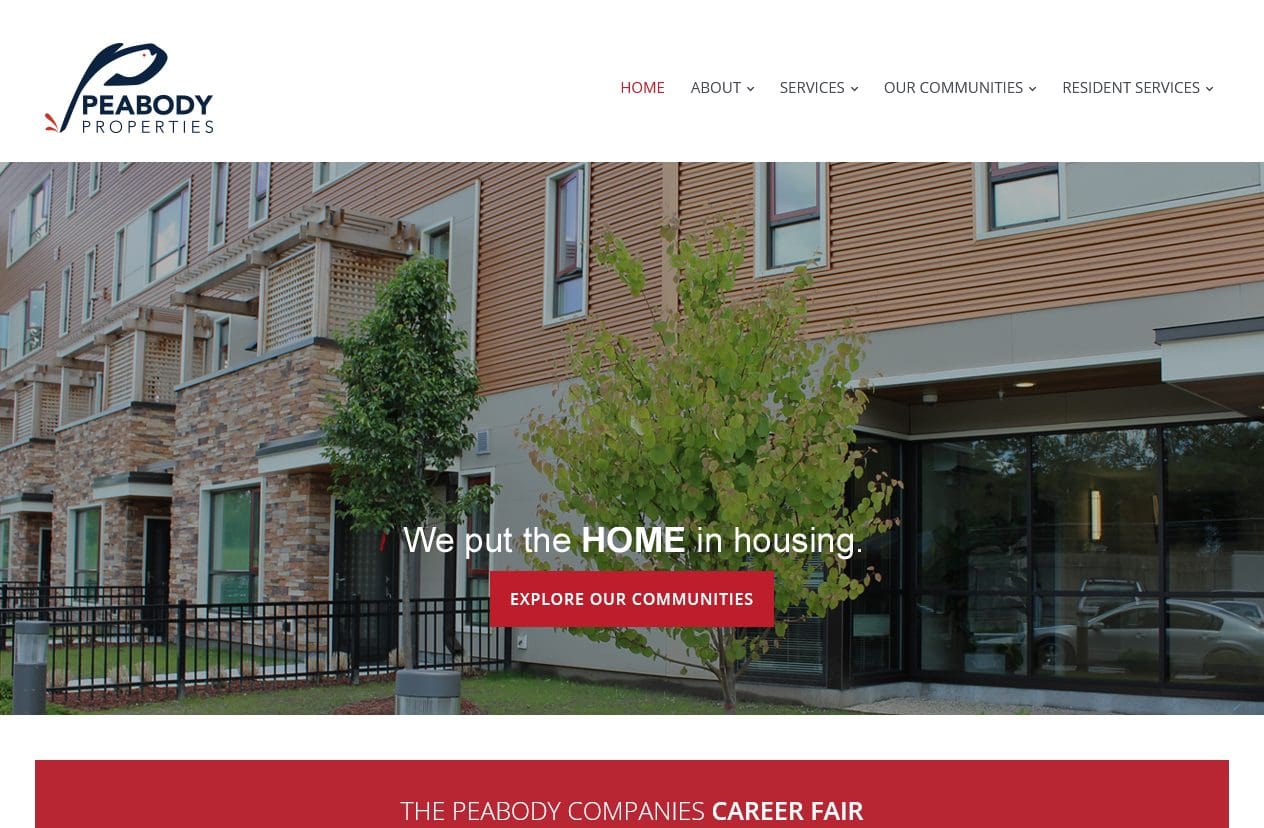The image depicts a webpage for Peabody Properties, featuring a clean, white background. In the upper left corner, there is a logo resembling a fish or a finger, accompanied by the text "Peabody Properties," with the name spelled out as P-E-A-B-O-D-Y. 

To the right of the logo, navigation tabs are displayed, including "Home," "About," "Services," "Our Communities," and "Resident Services." The tabs for "About," "Services," "Our Communities," and "Resident Services" feature downward arrows, indicating drop-down menus.

Below the navigation bar, there is an image of a brick apartment complex, complemented by trees and black fences in the foreground. The glass windows on the building reflect a car parked nearby. The bottom right corner of the image contains a text overlay with the phrase, "We put the 'home' in housing. Explore our communities." Additionally, at the bottom of the webpage, an announcement reads, "The Peabody Company's Career Fair."